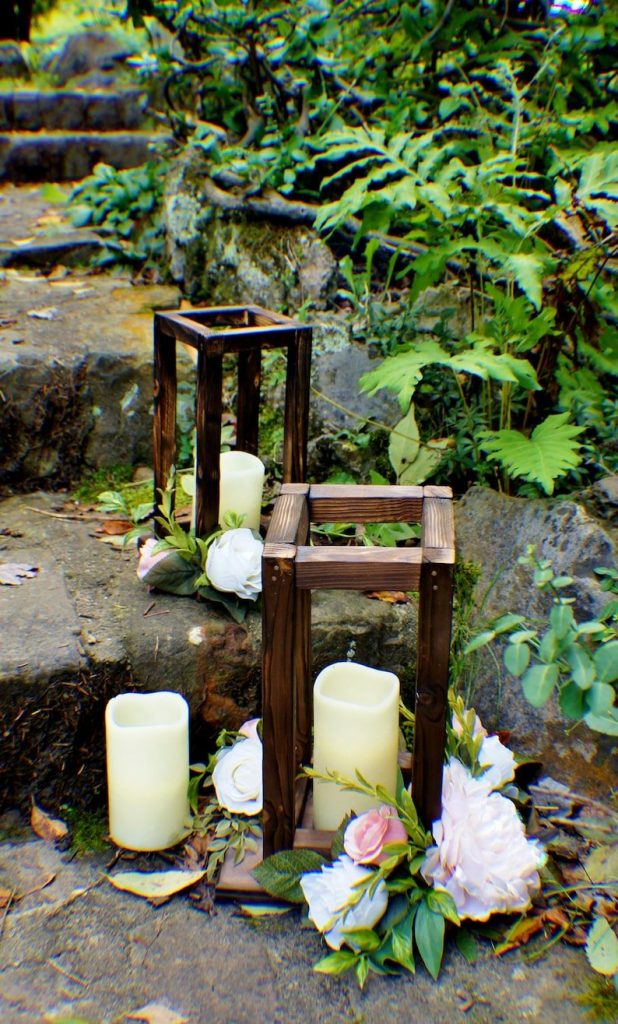This photograph captures a scene of a purposely staged display, set outdoors, likely in a natural or park-like environment. At the center, there are stone steps, smooth and seemingly carved directly from rock. On these steps, three large, off-white candles are prominently featured. Two of these candles are housed within wooden, rectangular frames that provide protection and stability. These frames are designed with an open square top. The candles, evidently used, are melted down to about halfway, with uneven tops and edges. The third candle, positioned to the left of the bottom-most framed candle, stands alone without any surrounding frame. 

Lush greenery, including ferns and various bushes, fills the right side of the image, adding a sense of natural beauty to the scene. Additionally, there are prominent white and pink flowers thoughtfully arranged around the steps, contributing to the staged aesthetic. A stick protrudes from the stones near the ferns, adding a touch of rustic charm. The overall ambiance suggests a tranquil setting, possibly along a path to a landmark or within a park, where open flames might typically be restricted. The meticulous placement of the candles and flowers emphasizes the intentional design of this serene corner.